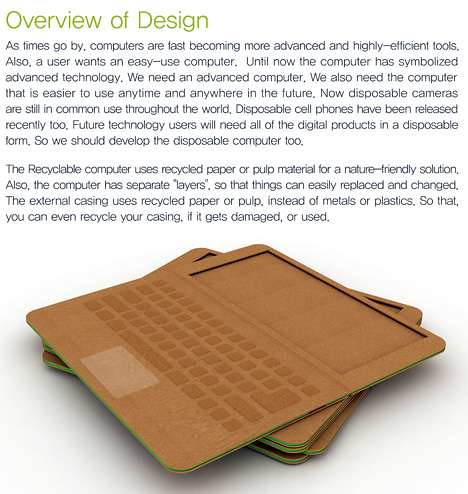The image is a conceptual advertisement or a screenshot of a web page detailing the design of an eco-friendly laptop made from recyclable materials. The laptop appears to be constructed from materials resembling felt or cardboard, with rounded corners for a sleek appearance. The upper half of the laptop features a wide, rectangular screen with green edges, while the lower half includes a keyboard and a trackpad, which looks somewhat like a coaster. 

In the upper left-hand corner of the image, green text reads "Overview of Design." Below this, in black text, the description explains how traditional computers have symbolized advanced technology but now there is a growing need for highly efficient and easy-to-use computers that can be utilized anytime and anywhere. The text discusses the evolution and common use of disposable cameras and cell phones, suggesting that future digital products, including computers, will need to be disposable as well. 

This recyclable computer uses recycled paper or pulp materials, offering a nature-friendly solution. The device has separate, replaceable layers, allowing for easy maintenance and updates. Its external casing made from recycled paper or pulp not only minimizes the use of metals or plastics but also allows the casing itself to be recycled if damaged or worn out.